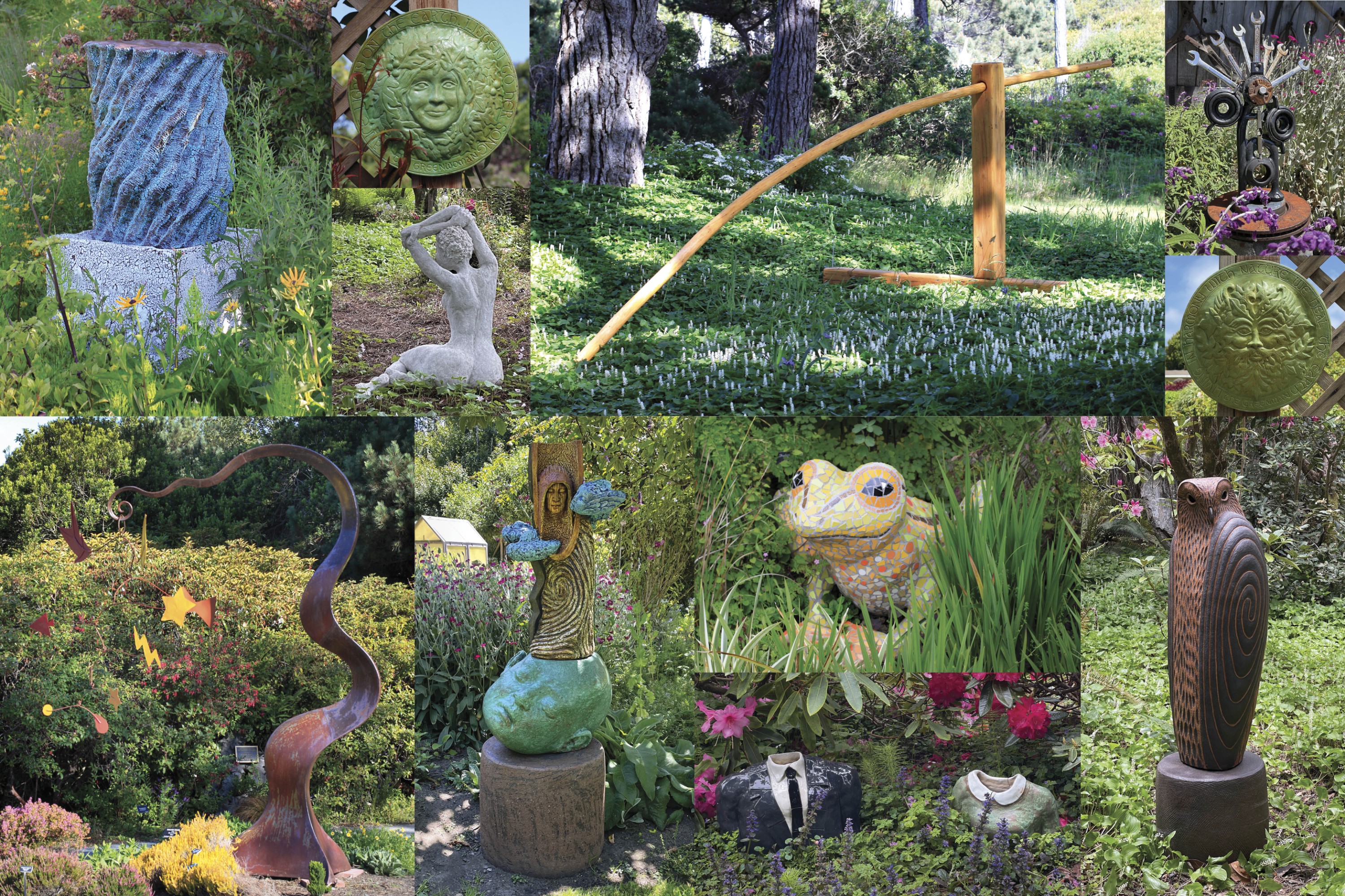The image features a collage of 8 to 10 rectangular photographs, arranged in two rows of four. Each photograph showcases a different section of a garden, all sharing the common element of grass-covered ground. The garden scenes feature various interesting sculptures and decorations. Among them, there's a stone statue of a frog, an owl placed on the ground, and a sitting woman. One photo captures a unique abstract sculpture resembling a wave floating upwards. Another image depicts a wooden contraption looking like a four-post structure with a round pole. There's also a distinctive statue that seems to integrate elements resembling a fire hydrant and wrenches, along with a headless couple emerging from the ground. Additionally, the top left photograph showcases a spiral concrete sculpture, and nearby is a green ceramic disc adorned with a woman's face surrounded by a wreath. The setup highlights a variety of creative and artistic garden ornaments, making the garden eclectic and visually engaging.